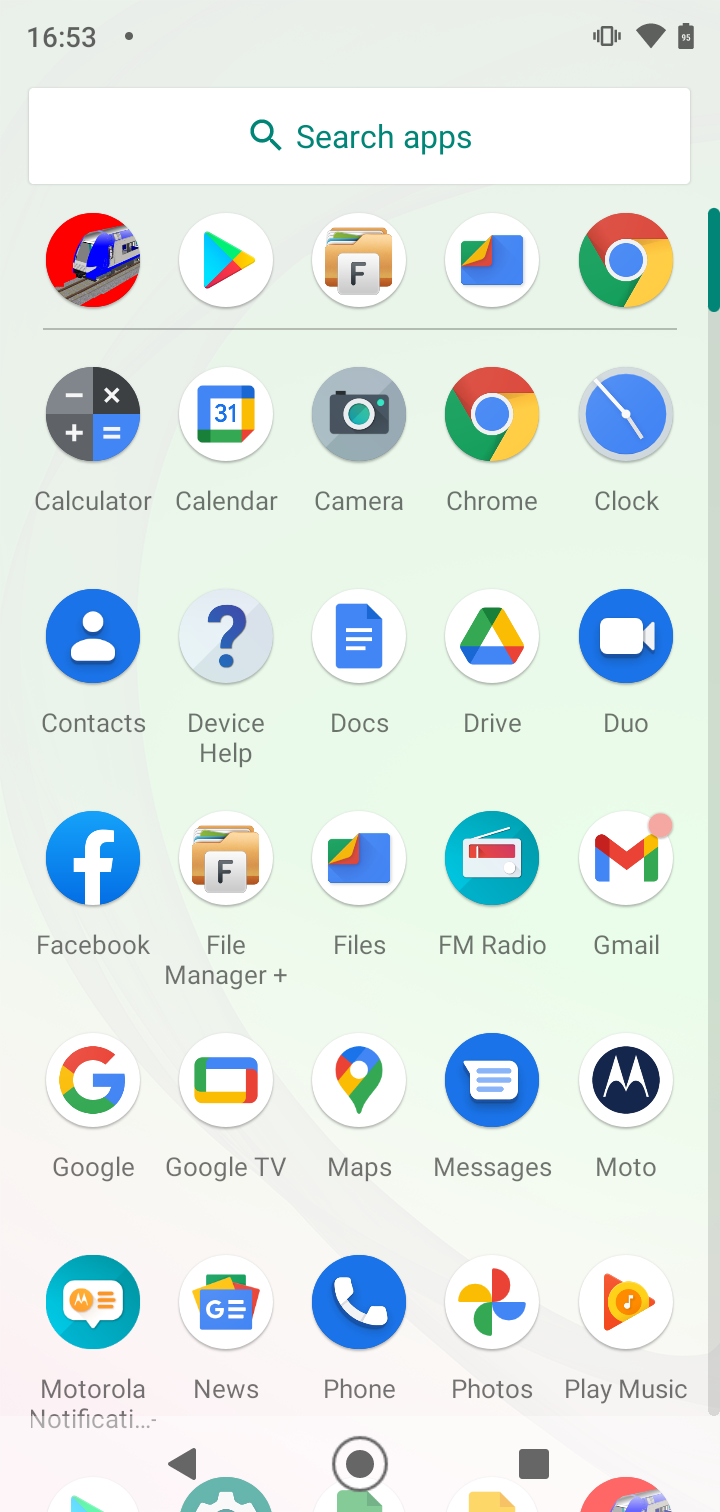The image displays a screen densely packed with various icons, reminiscent of a smartphone's home screen, yet distinct due to a search field labeled "Search apps" located at the top. In the upper left corner, there's a timestamp, while the upper right corner features indicators for Wi-Fi, battery status, and an unidentified icon. 

The icon layout begins with an unlabeled row, presumably consisting of frequently used apps like Chrome. This row includes five icons that interchangeably cover navigation, utilities, and system essentials. 

Below this, several labeled rows organize the apps systematically:

1. **Top row (Unlabeled):** Recognizable icons such as Chrome and other familiar app symbols, though specifics are somewhat unclear.
   
2. **First labeled row:** 
   - Calculator
   - Calendar
   - Camera
   - Chrome
   - Clock

3. **Second labeled row:**
   - Contacts
   - Device Help
   - Docs
   - Drive
   - Duo

4. **Third labeled row:**
   - Facebook
   - File Manager
   - Files
   - FM Radio
   - Gmail

5. **Fourth labeled row:**
   - Google
   - Google TV
   - Maps
   - Messages
   - Moto

6. **Fifth labeled row:**
   - Motorola Notification
   - News
   - Phone
   - Photos
   - Play Music

7. **Sixth row (partially visible):** Only the top halves of the icons are seen, with no labels visible.

This meticulously laid-out interface suggests a highly organized digital environment, designed for efficient access to a myriad of applications. The screen's specific details, from the search bar to the discrete indicators, provide a clear snapshot of a tech-savvy user's app management system.